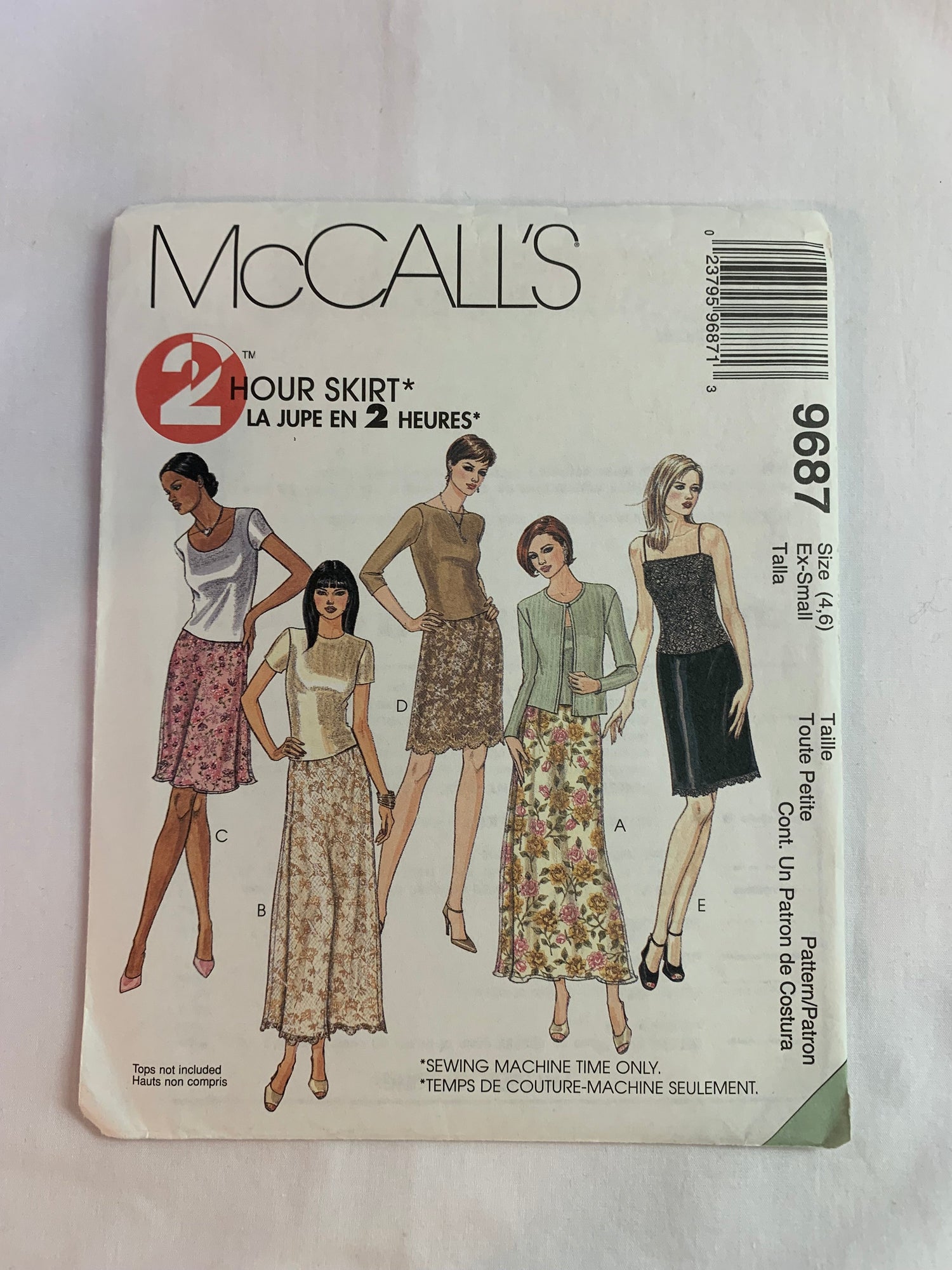This image features the cover of a McCall's pattern package, specifically McCall's Pattern 9687. The cover showcases a series of artistic illustrations of young women dressed in stylish skirts, each differing in length and design, paired with various tops. At the top of the package, "McCall's" is boldly displayed, followed by the phrase "Tour Jupe" (To Our Skirt) in French. Directly below this, it emphasizes that tops are not included, again with the French translation provided. The text "sewing machine time only" appears underneath, in both English and French ("temps"). The pattern number "9687" is prominently written in vertical letters along the right side of the package. Additional details regarding the pattern sizes and a barcode are located at the top right corner of the cover. The fashionable attire depicted in the illustrations highlights a variety of elegant and trendy skirt styles, making this pattern an appealing option for fashion enthusiasts and sewers alike.